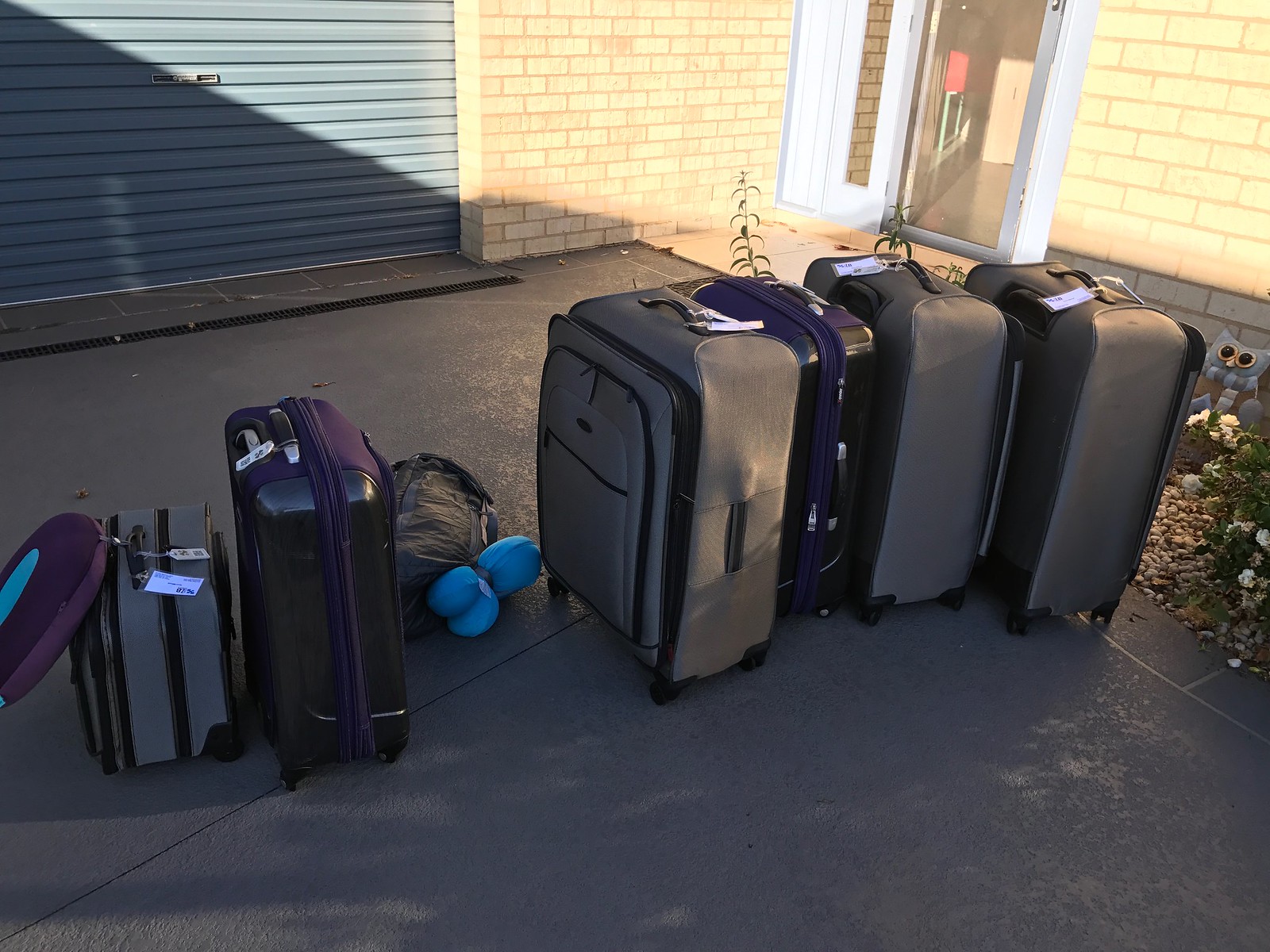In this image set outside of a light-yellow brick house, a row of six upright suitcases and one black duffel bag are neatly lined up in a driveway. The suitcases are of varying sizes, suggesting they belong to a family that has just returned from a lengthy trip. To the left of the scene, a medium-blue closed garage door forms part of the backdrop, while to the right corner, a glass storm door with white borders stands near a small garden area that features rocks, plants, flowers, and an owl figurine. The suitcases themselves include three large metallic gray fabric cases, two shiny purple ones, and a smaller gray one. Each piece of luggage has its handle extended and a white tag attached at the top. Among the suitcases, near the lower middle left, a few bright blue objects, perhaps shoes or slippers, catch the eye, suggesting they are packed or slipped between the bags. The scene captures a moment that feels like the calm after a lengthy journey.